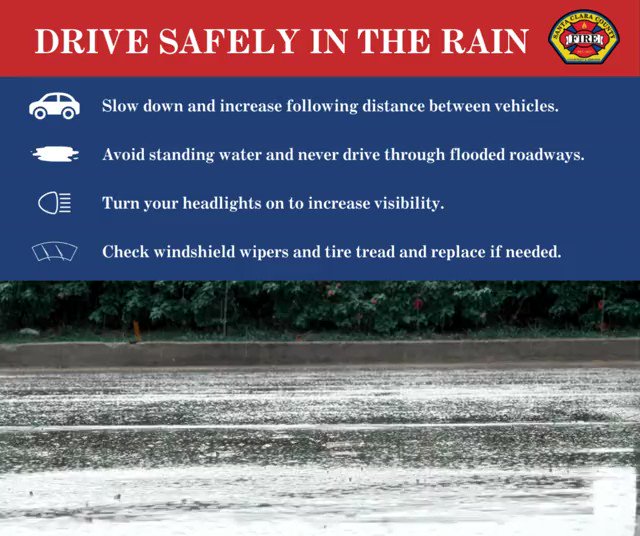This image is a public service announcement from the Santa Clara County Fire Department, advising drivers to exercise caution while driving in rainy conditions. The top of the PSA features a red-bordered title, "Drive Safely in the Rain," accompanied by the Santa Clara County Fire Department badge in the upper right corner. Below the title, essential safety tips are provided within a blue block. These include: slowing down and increasing the following distance between vehicles, avoiding standing water, never driving through flooded roadways, turning on headlights to improve visibility, and checking windshield wipers and tire tread, replacing them if necessary. These tips are illustrated with corresponding images: a car, a puddle, a headlight, and windshield wipers. The bottom section of the PSA displays a photograph of a wet roadway, reinforcing the message to be cautious on slick surfaces.